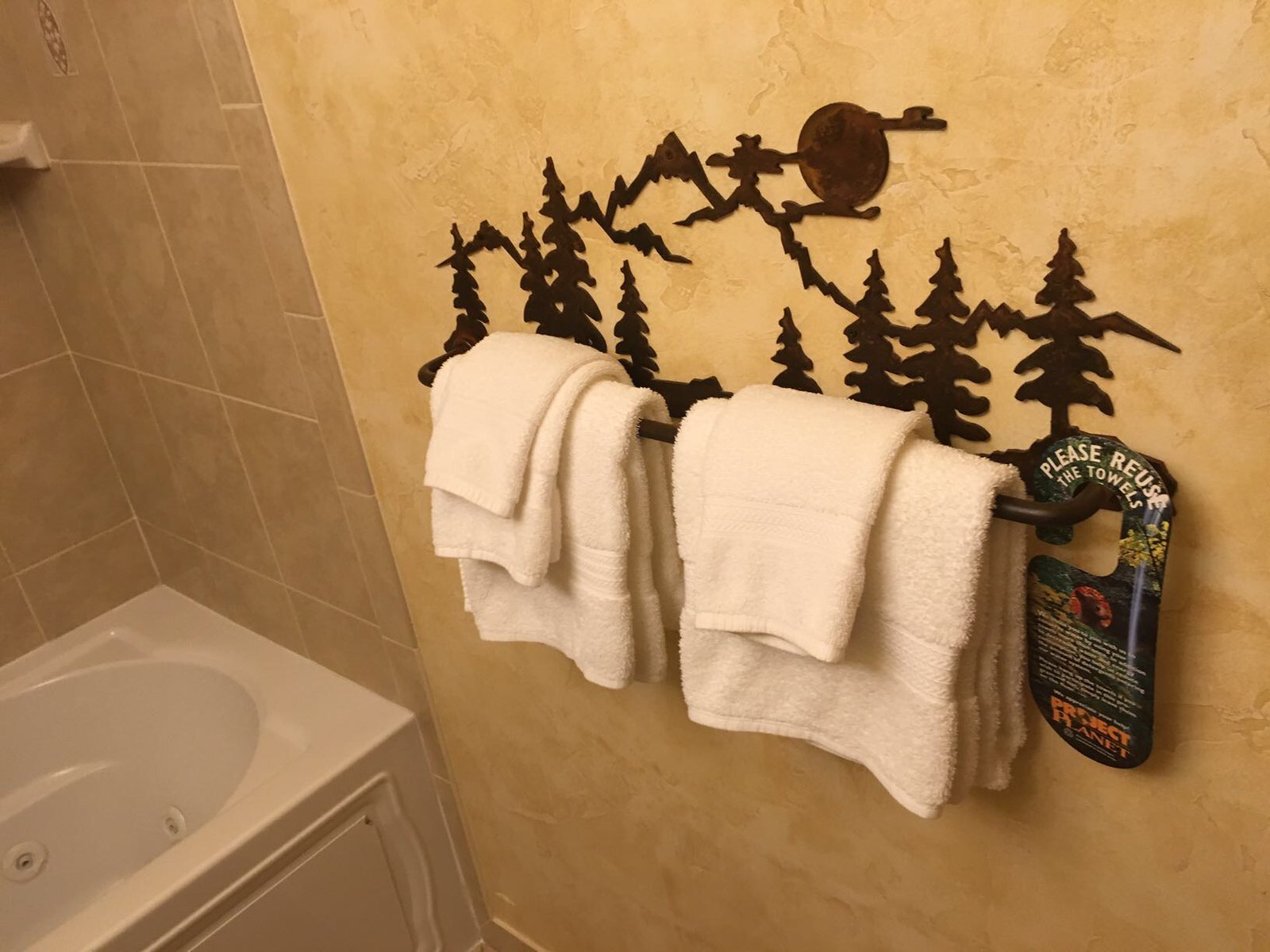This image captures a hotel bathroom with a detailed and cozy ambiance. Central in the frame is a brown towel bar mounted on a textured light brown wall adorned with an illustration of mountains, trees, and the moon. Neatly folded on the towel bar are multiple white towels, including both hand towels and at least one body towel. To the right of the towel bar hangs a small sign that reads "Please reuse the towels," with additional text below that states "Project Planet." Toward the left side of the image, a portion of a white bathtub with hot tub jets and etched lines in its paneling is visible, along with some of the surrounding beige-tiled wall. The overall color scheme of the bathroom is warm hues of brown, tan, and beige, and there's no shower curtain in sight.